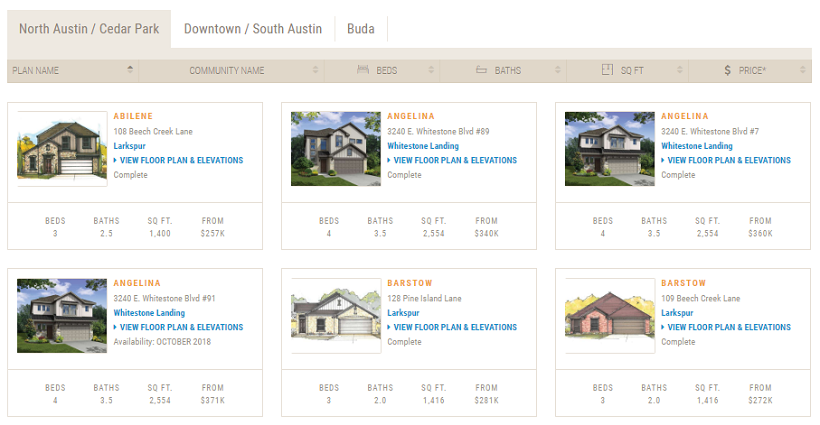This image is a detailed screenshot from a real estate website, most likely for a custom home builder. The top of the image features a navigational menu with three options: "North Austin / Cedar Park" is highlighted on a beige background, indicating it is the selected tab, while "Downtown / South Austin" and "Buda" are displayed on a white background. Below this menu, the page outlines various home plans with categories labeled "Plan Name," "Community Name," "Beds," "Baths," "Square Feet," and "Price" on a beige background.

Under this header, six artistic renderings of homes are displayed against a white background. These renderings include names written in orange: from left to right, "Abilene," "Angelina," "Angelina," and "Barstow." The first two sets display two-story homes, while the "Barstow" homes are noted as one-story designs. Each rendering has a clickable link labeled "View Floor Plan and Elevations," which provides additional details.

Underneath each home rendering, the specifications such as the number of beds, baths, square footage, and price range are listed. Prices vary, with the least expensive option starting at $257,000 and the most expensive beginning at $360,000.